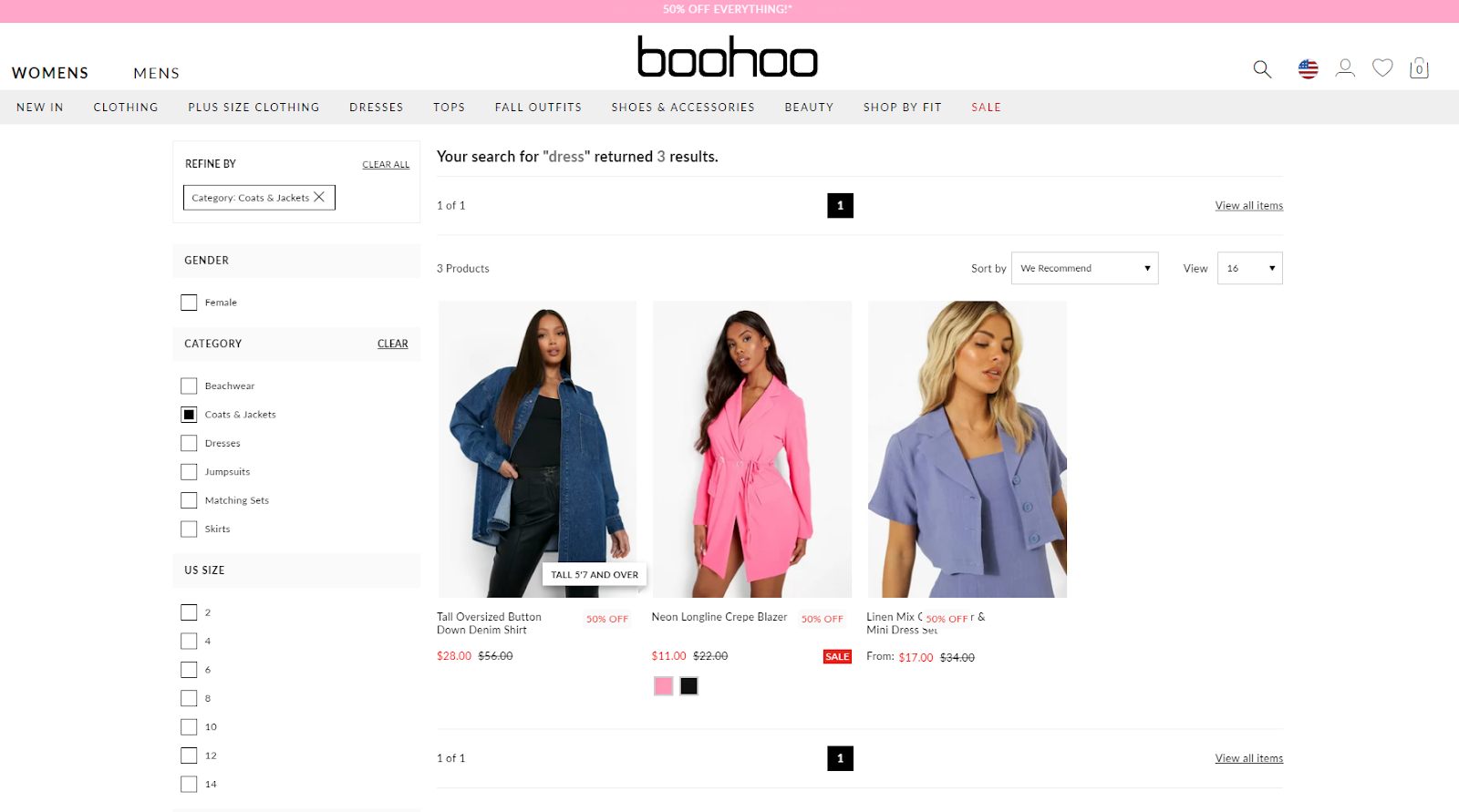The top of the image features a women's website banner with a pink bar displaying a promotion: "50% off Everything*" (with asterisks indicating stipulations). Below the banner, there are separate navigational tabs for "Women's" and "Men's" sections, with the "Women's" tab highlighted in black to indicate its selection.

The main section of the page shows three women posing, each highlighting a different product. 

1. The first woman, a black woman, wears a long button-down denim shirt that is open. She has her right hand on her hip with her other arm down. Her hair is styled to her right, partially covering her jacket. Underneath, she wears a black tank top paired with black pants and a belt. This outfit is listed as a "Tall Oversized Button-Down," currently on sale for 50% off, marked down from $56 to $28.

2. The middle model, also a black woman, is dressed in a pink button-up blazer with long hair flowing down. This blazer is available in both pink and black color options. It is also on sale, reduced from $22 to $11, with the sale price highlighted in red.

3. To the far right is a woman dressed in a blue top and matching blue dress. The price for this dress has been halved from $34 to $17.

Above the product listings, there's a functionality to sort the items through a drop-down box and adjust the view preferences. Additionally, on the left sidebar, there is a "Refine By" column allowing shoppers to filter options by gender (with a checkbox for 'Female'), categories (Beachwear, Coats and Jackets, Dresses, Jumpsuits, Matching Sets, and Skirts), and US sizes.